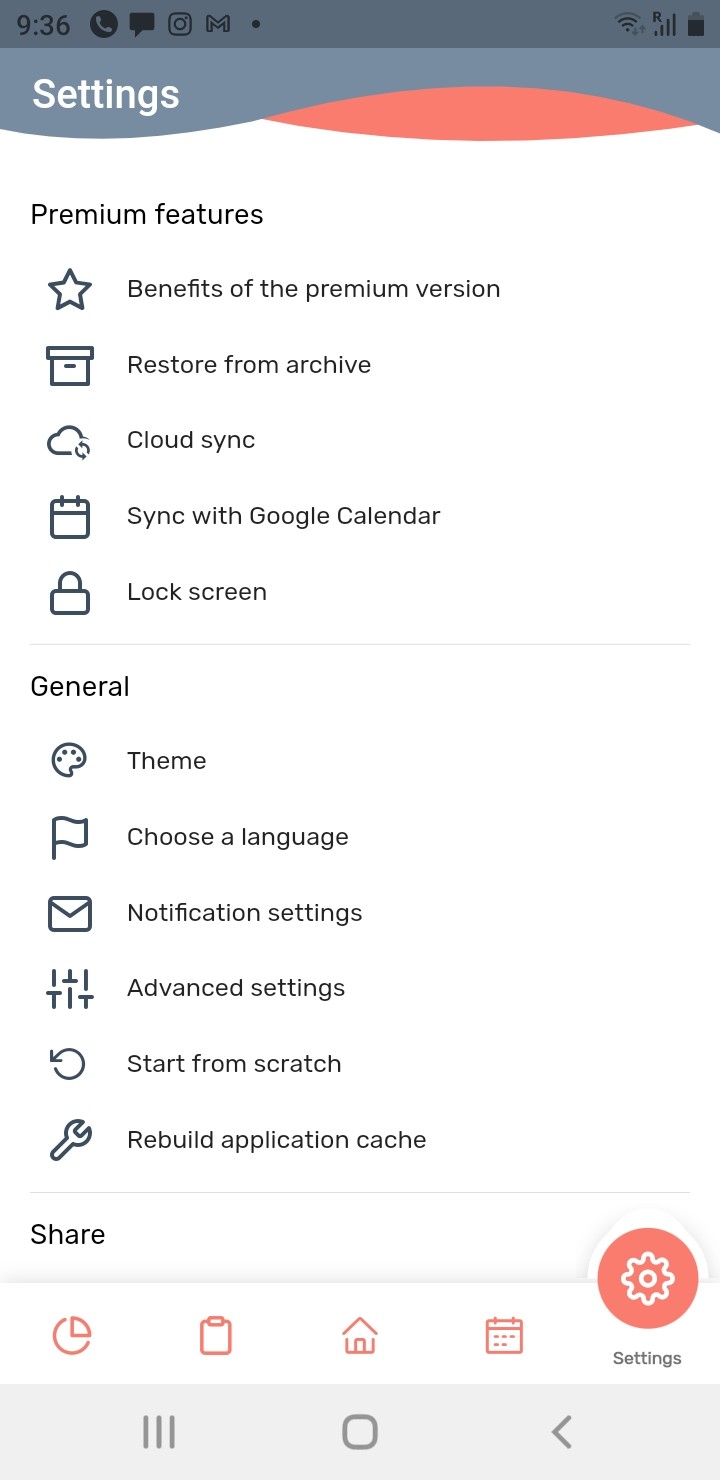The image depicts a settings screen from a cell phone, identifiable by the standard battery, signal strength, and other status icons located in the upper right-hand corner, and the time displayed in the upper left-hand corner. Surrounding these elements is a gray rectangular bar.

Beneath this bar, there is another rectangular area with an artistic blend of shades—gray and peach. In the center of this section, the word "Settings" is displayed in white letters.

Further down, the screen is divided into two sections: Premium Features and General Features. The Premium Features section lists options with accompanying icons and brief descriptions. The first item is marked by a star icon and reads "Benefits of the Premium Version," followed by four additional premium features.

The General Features section also includes icons next to each option. For example, a wrench icon accompanies the option to "Rebuild Application Cache," and an envelope icon is for notification settings. At the very bottom of the screen, there are various hyperlink buttons to navigate to different parts of the settings menu, reflecting the expansive and detailed nature of cell phone settings.